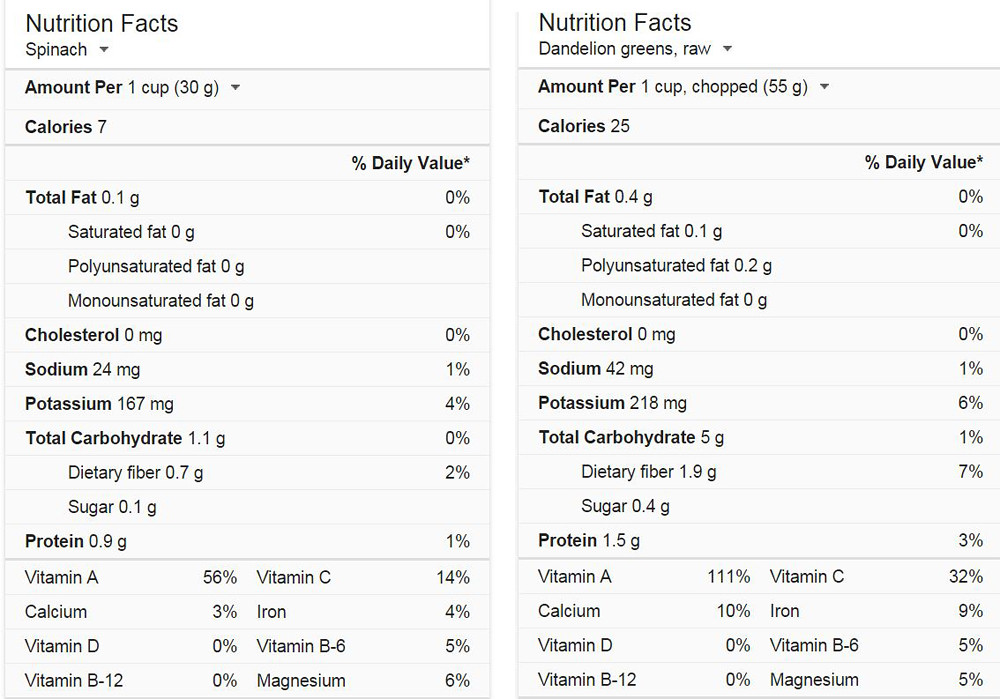The image displays two distinct nutrition facts labels, each devoid of associated product imagery. On the left, the label pertains to spinach, revealing that one cup contains 7 calories. Key nutritional details include 24 milligrams of sodium, 167 milligrams of potassium, 1.1 grams of total carbohydrates, 0.7 grams of dietary fiber, 0.9 grams of protein, and 56% of the daily recommended intake of vitamin A. Conversely, the label on the right details the nutrition facts for raw dandelion greens. One cup of these greens provides 25 calories, 42 milligrams of sodium, 218 milligrams of potassium, 5 grams of total carbohydrates, 1.9 grams of dietary fiber, 1.5 grams of protein, and a striking 111% of the daily recommended intake of vitamin A.